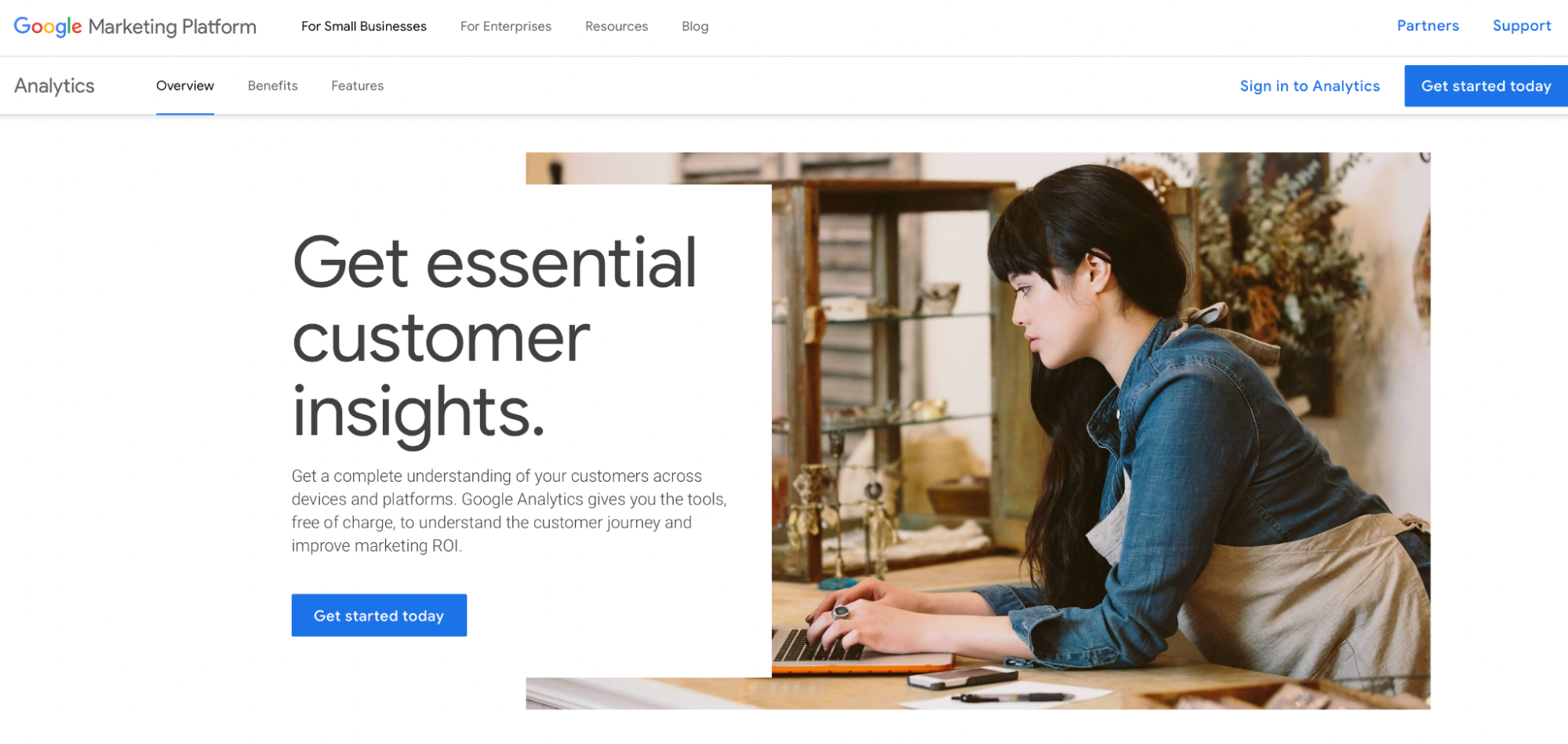In this image, a Google Analytics webpage is displayed prominently. At the top left corner, the iconic Google logo is visible in its classic blue, red, yellow, and green colors. Below the logo, various navigation options are listed, including "Marketing Platform," "For Small Businesses," "For Enterprises," "Resources," "Blog," "Analytics," "Overview," "Benefits," and "Features." The text on the page emphasizes the utility of Google Analytics, highlighting its capability to provide essential customer insights and a comprehensive understanding of customer behavior across multiple devices and platforms. It mentions that Google Analytics tools are available for free to help improve marketing ROI, with prompts to "Get started today."

In the top right corner, additional links such as "Partners," "Support," and "Sign In to Analytics" are available. The foreground of the image features a woman typing on a laptop. She is dressed in a brown apron and a blue jacket, suggesting she might be a small business owner or someone working in a hands-on environment. A neatly arranged table surrounds her, featuring a flower, a mobile device, and a pen, adding a touch of daily life and professionalism to the scene.